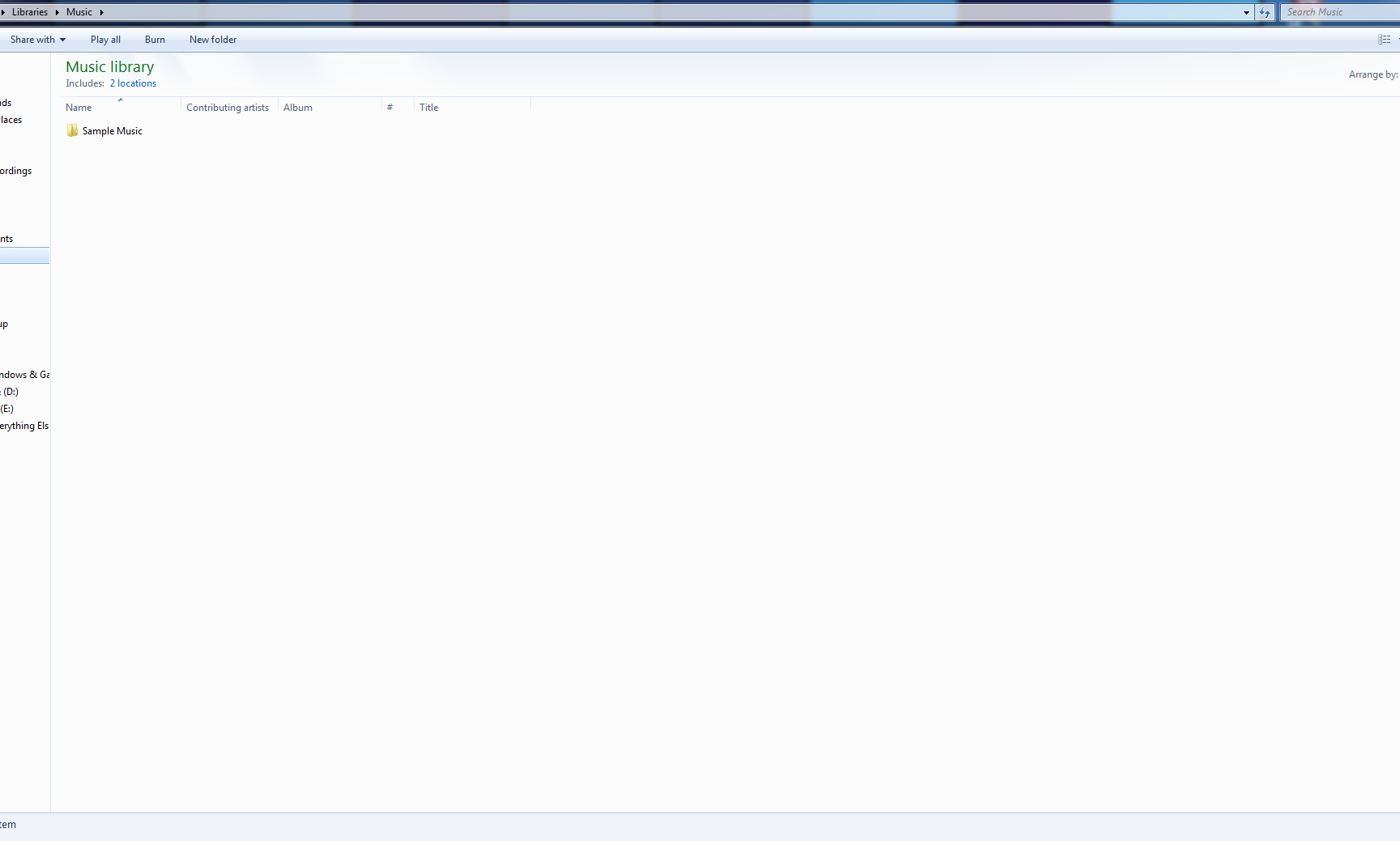The screenshot showcases a user interface from what appears to be a CD or DVD burning application, rendered in a simplistic and somewhat low-quality design. At the top, a blue navigation bar is present. In the upper left corner, breadcrumb navigation labeled "Libraries > Music" is visible, indicating the user's current directory within the application. On the upper right side of this blue bar, a search field with the placeholder text "Search Music" is situated, allowing users to look up specific music files.

Directly below the navigation bar, there's a light blue toolbar offering several options: "Share with us," "Play all," "Burn," "New folder," among other commands, although some of the options are difficult to read clearly. 

The main section of the screen displays the heading "Music Library" in red font, which notes that the library includes content from two locations. Below this heading, the content is organized in a spreadsheet-like format with columns labeled "Name," "Contributing Artists," "Album," and "Title."

A folder icon resembling a manila folder labeled "Sample Music" is visible within this layout, signifying a directory that may contain sample music files.

Additionally, a partially visible menu is located on the left side of the screen, although it is not fully legible. In the upper right corner of the main section, an option to "Arrange by" various file attributes is provided for sorting the displayed content. 

Overall, the application's interface appears basic and functional, designed for managing and burning music files to CDs or DVDs.